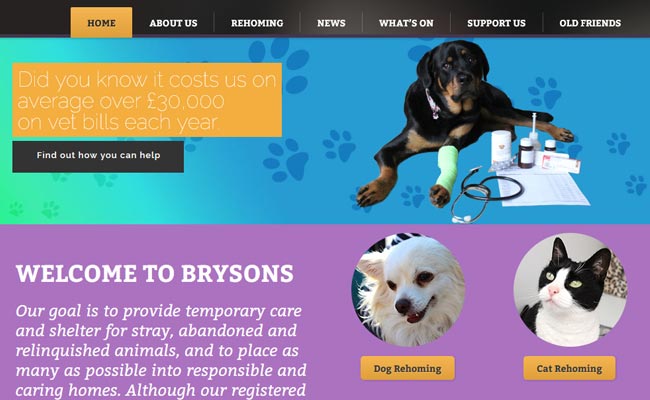The website immediately projects its focus on animal welfare through a prominently featured image of a black dog. This dog has distinctive tan markings on his chin, nose, and paws, and is laying down with a green cast on his left paw. He wears a collar and rests next to a stethoscope and a piece of paper topped with images of medicine bottles. In the left corner, a text note mentions that the organization spends over €30,000 annually on veterinary bills.

At the top of the site, a black header contains navigational links: "Home," "About Us," "Rehoming," "News," "What's On," "Support Us," and "Old Friends." The "Home" link is highlighted in orange, indicating the current page. Below the header, a black box underneath an orange one invites visitors to "find out how you can help." 

The page's lower half has a purple background and welcomes visitors to Bryson's, outlining its mission to provide temporary care and shelter for stray, abandoned, and relinquished animals, aiming to place as many of them as possible into caring homes. The text cuts off with, "A low R registered," and below this is a picture of a beautiful white dog labeled "Dog Rehoming" next to a black and white cat labeled "Cat Rehoming," both signs marked in orange.